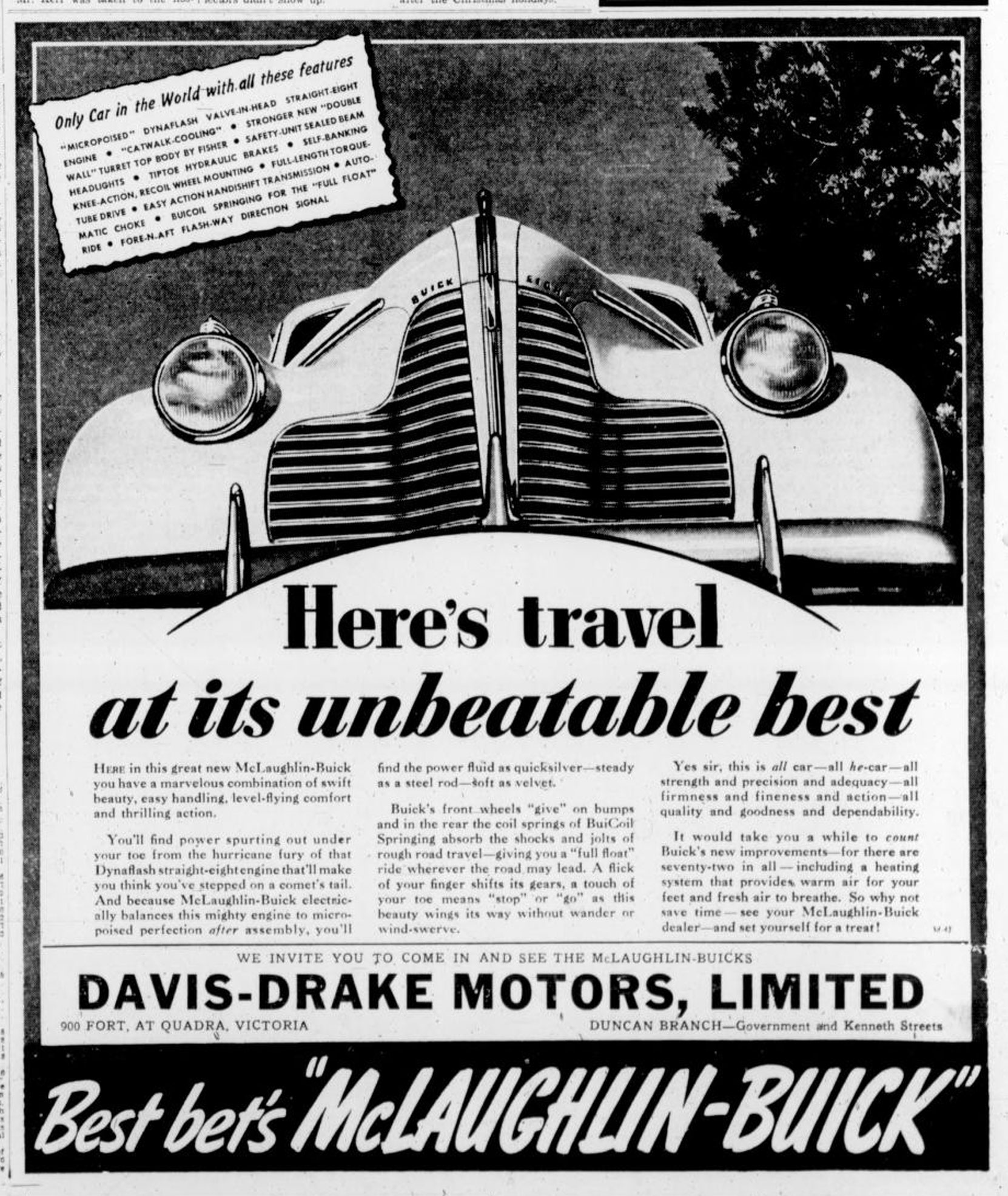This vintage advertisement for the classic Buick Regal, scanned from its original black and white print, showcases a commanding perspective of the car’s front end. The image, which occupies the top third to half of the page, features an eye-catching illustration of the grille and round headlights from a lower angle, emphasizing the vehicle’s high-peaked hood. Below this striking visual, bold black text announces, “Here’s travel at its unbeatable best,” emphasizing the unparalleled driving experience offered by the Buick.

Underneath, three columns of black text expound on the Buick's remarkable features and performance. The detailed article extols the virtues of the McLaughlin Buick, highlighting its swift beauty, easy handling, and level-flying comfort. It praises the thrilling action and power of its Dynaflash straight-eight engine, noted for its fluidity, steadiness, and velvet softness thanks to the micro-poised perfection achieved post-assembly. The advertisement further describes the front end’s responsiveness to bumps and the rear coil spring's ability to absorb shocks for a smooth ride. It emphasizes the convenience of finger-flick gear shifts and toe-touch brakes that ensure seamless driving.

Additionally, the advertisement mentions the myriad of 72 new improvements, including a sophisticated heating system that provides warm air for the feet and fresh air for breathing. The concluding invitation encourages potential buyers to visit their local McLaughlin Buick dealer to experience the car firsthand.

The ad is punctuated by the branding of Davis-Drake Motors Limited, along with their addresses in Victoria and Duncan. At the bottom, a handwritten-style text on a black background proudly proclaims, “Best Bets, McLaughlin Buick,” rounding off an advertisement that captures both the elegance and engineering marvel of the era’s Buick Regal.